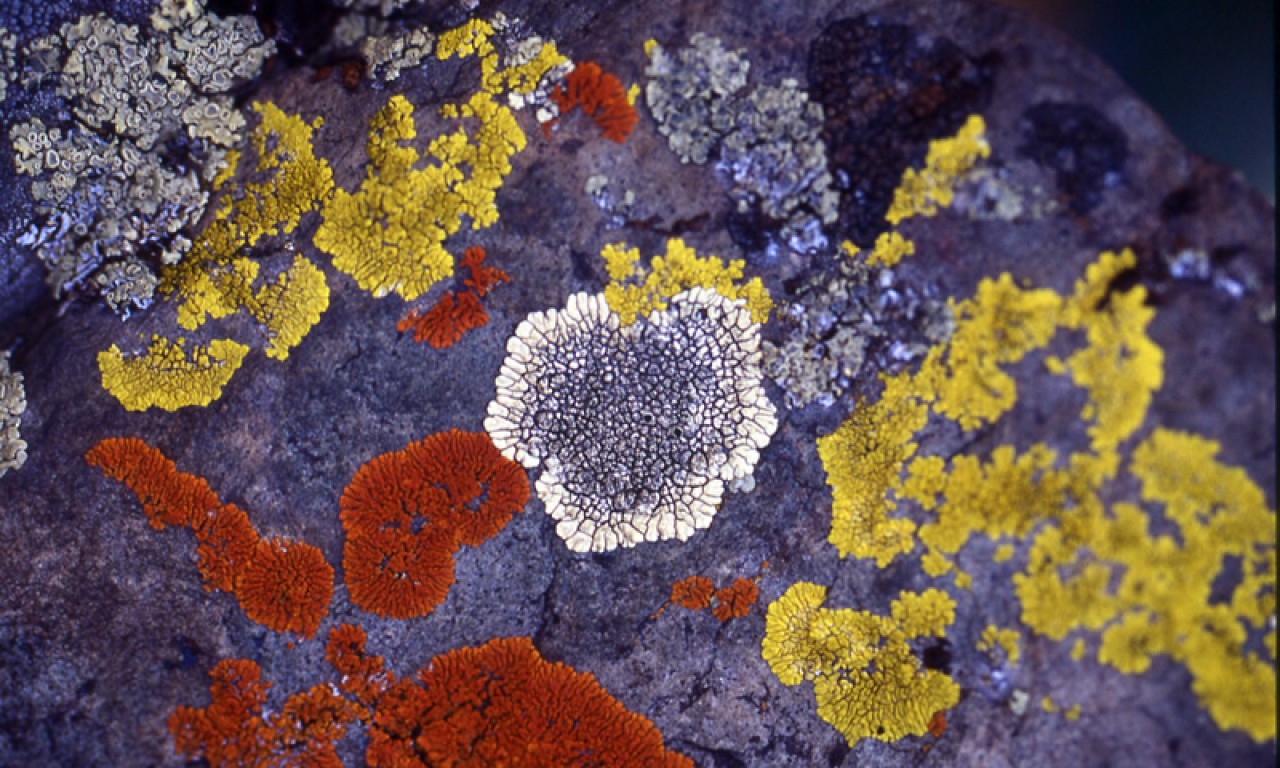The photograph, a color image in landscape orientation, captures a detailed underwater scene of algae, lichen, and mold-like growths on gray rocks. Dominating the center is an oval-shaped lichen with a white border and a blue center, accented by radiating black lines resembling teeth. Surrounding this central cluster, lighter gray rocks with a mottled dark brown to cream surface host several scattered patches. To the lower left, there are bright rusty red clusters, their flaky textures partially breaking apart. Nearby, the bottom right boasts some out-of-focus, dirty yellow formations. The upper right corner of the photo is home to darker rocks, including a heart-shaped section that's nearly black. Additionally, golden ochre lichen patches are prevalent on the right side and are interspersed throughout the top left corner, creating a visually engaging composition of natural earthy hues and intricate textures.